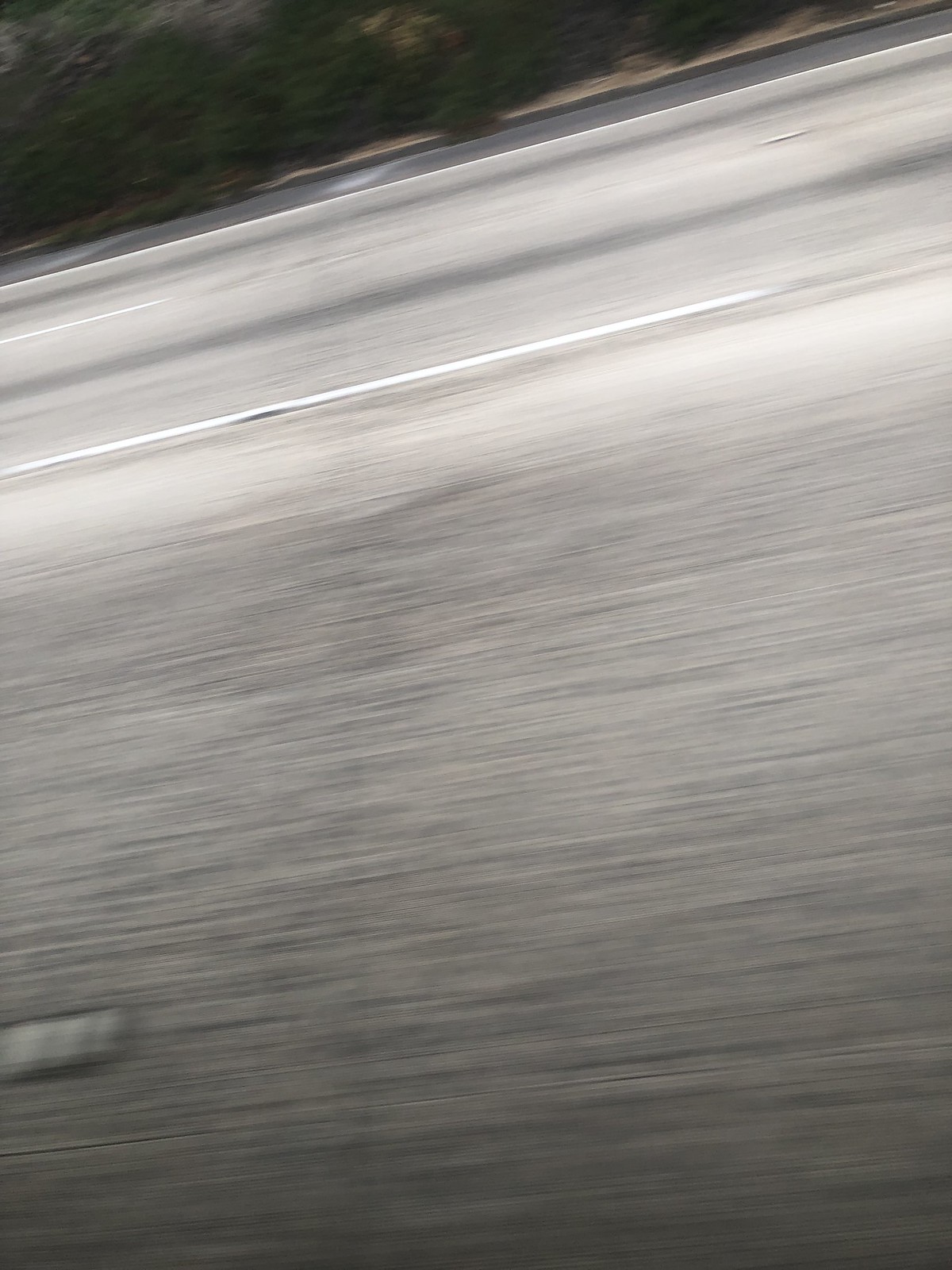The image depicts a blurred, real-life scene captured from a moving vehicle. The main subject of the photo is a gray asphalt road with distinct white markings: a solid white stripe and a dotted line, likely representing lane separators. The blurriness suggests motion from left to right, with streaks of black, gray, and white accentuating the sense of speed. The lower two-thirds of the image are dominated by the road's surface, which varies in shades of gray and black. Alongside the road, there is a strip of white paint and lighter gray areas. The upper portion of the image reveals an incline or hillside lined with greenery, including bushes and patches of brown dirt, contributing to the impression of a roadside embankment. This combination of visual cues, though indistinct due to the blurriness, creates a dynamic scene of a road bordered by natural elements.